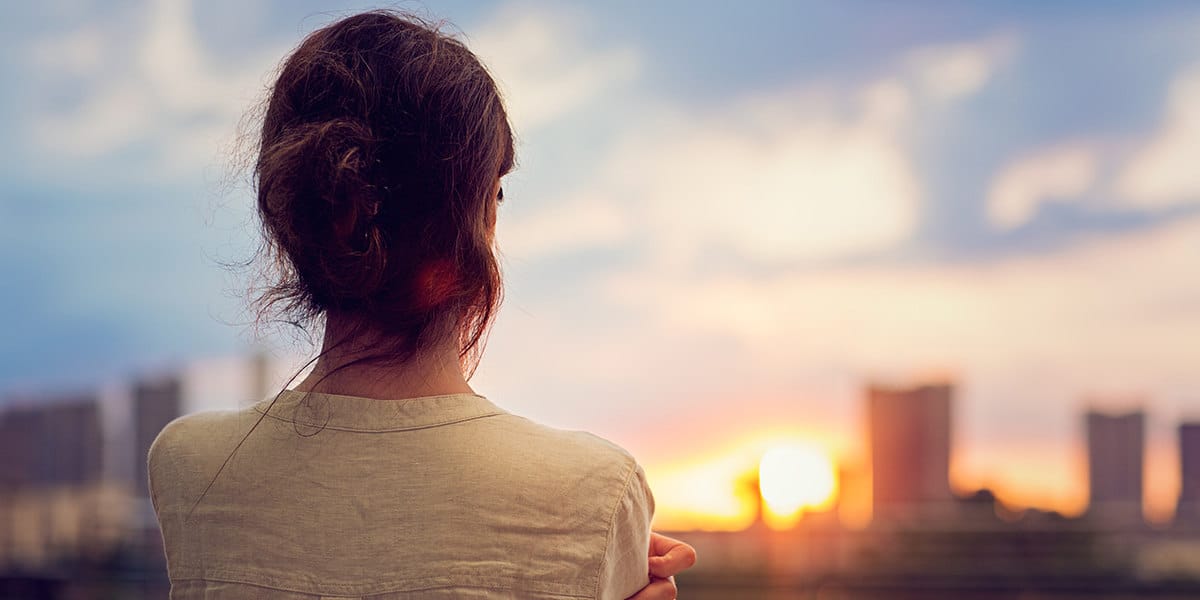In the image, we see the back of a woman’s head and shoulders as she gazes out over a cityscape at dawn. Her brown hair is pulled up and clipped at the back of her head, with a few strands appearing slightly disheveled on the right side. She wears a wrinkled, collarless white blouse, and her left arm is crossed over her chest, with her fingers resting on her right shoulder. The photograph captures a serene blue sky adorned with white clouds and the rising sun, which paints the horizon with vibrant hues of orange, yellow, and white. The cityscape features tall buildings that span both the left and right sides of the image, though much of the background is softly out of focus. The rectangular, horizontal composition emphasizes the tranquil moment of contemplation as the woman observes the awakening city below.